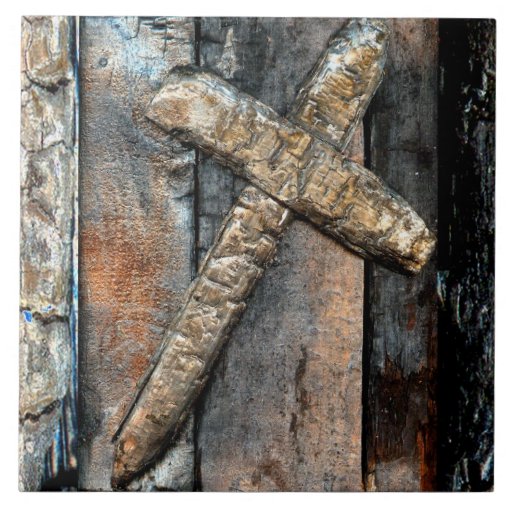This square photograph, despite its modest quality, captures an outdoor scene bathed in bright natural light, showcasing a rustic wooden wall made from rough-hewn planks. The wall features a variety of colors, ranging from grays and rusty browns to pale browns, all sealed with a clear varnish that adds a subtle shine. Superimposed on this wooden backdrop is a weathered cross, slightly tilted to the right. The cross, made from a mix of wood and possibly tarnished metal, exhibits a blend of beige, gray, brown, and hints of red, enhancing its antiquated appearance. This central cross, with a longer vertical line tapering to a pointed bottom, connects the image elements, creating a cohesive yet rugged visual experience. The overall ambiance hints at an old wooden structure, possibly located in a forest, adding to the scene's rustic charm.